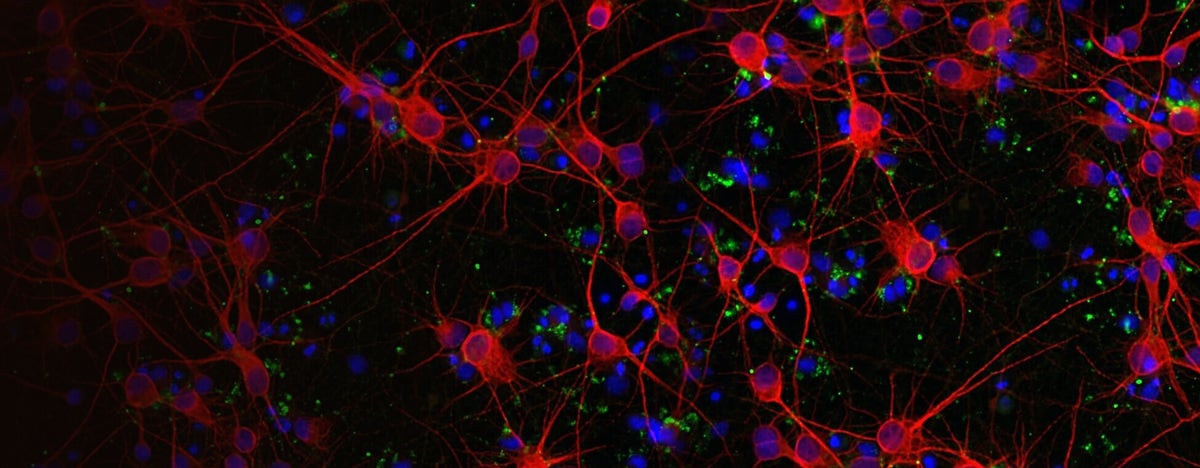The image displays a large black rectangular canvas filled with vibrant and intricate details. Predominantly, it features a myriad of red lines and dots that create a striking visual against the dark background. These red elements are interconnected, with lines stretching from dot to dot. Blue dots of varying sizes, some appearing as small blotches, are scattered throughout, contributing to the image's complex texture. Green hues, reminiscent of neon lights, subtly accent the backdrop. The left side of the image is notably darker, making details there less distinguishable. Overall, the image resembles something observed under a microscope, teeming with colors—primarily red, blue, and green—illuminated against a black background, creating a visually compelling and highly detailed composition.